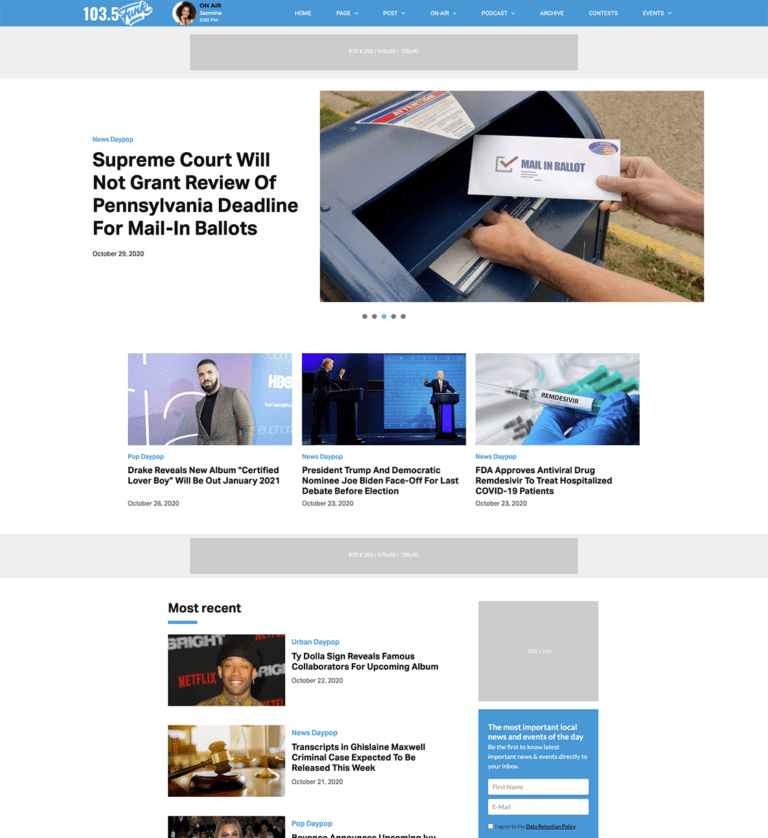The website for 103.5 Funk features a prominent header that might initially be mistaken for an official United States Post Office site due to its emphasis on voting. It includes an image of someone depositing a mail-in ballot into a public mailbox, reinforcing the voting theme. The page, zoomed in at 200%, reveals a headline stating, "Supreme Court will not grant review of Pennsylvania deadline for mail-in ballots."

Below this main focus, the website is divided into sections with various images and updates. On one side, there's a picture of Drake announcing his new album. Next to it, there are images from a debate between Joe Biden and Donald Trump. Another image highlights the FDA's recent approval of an antiviral drug.

Further down, in a section dedicated to recent updates, the site presents a collection of the latest news articles and developments.